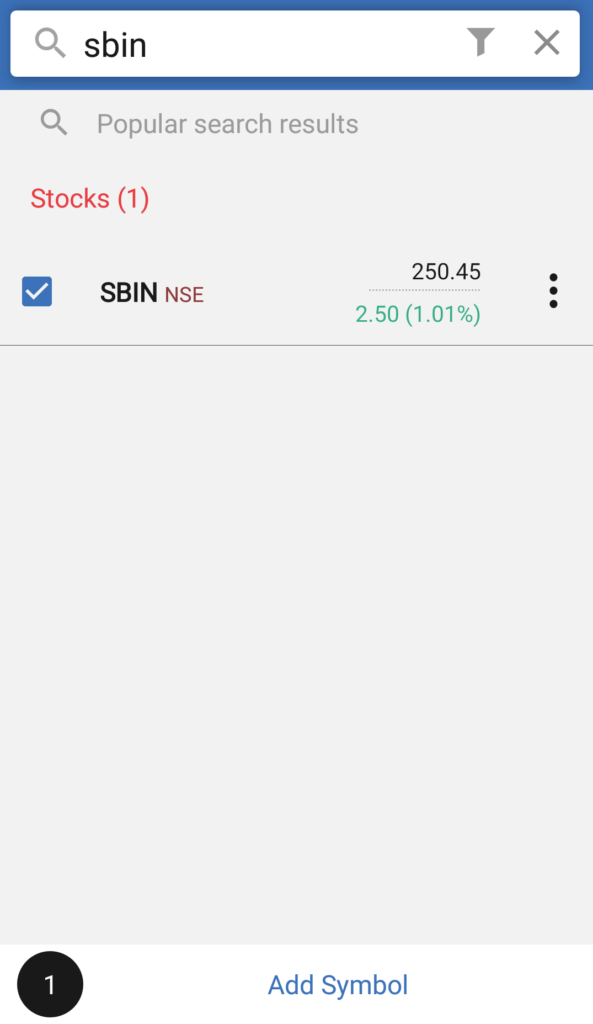This mobile screenshot showcases a stock trading app interface. At the top, there's a prominent search bar featuring a small magnifying glass icon on the left to initiate searches, currently displaying the text "Espen". To the right of the search bar, there's a filter icon resembling a funnel, allowing users to refine search options. Adjacent to that is a gray 'X' icon, providing an easy way to clear the search field, which is particularly useful on mobile devices.

Below the search bar, the heading "Popular Search Results" is displayed alongside a search icon, indicating either a list of popular searches or a reference to the single search result below. The result shows "Espen NSE" with the category "stocks". This suggests that the app specializes in stock information and possibly trading.

Towards the bottom left of the screen, a black circle with a white number '1' is present, accompanied by a blue "Add Symbol" button, facilitating the addition of new stock symbols to the user's watchlist. Below these elements, the stock details for Espen NSE are shown, including a price listed as $250.45 and additional figures: $2.5 and 1.01%. These may represent price changes or percentage shifts, providing comprehensive financial metrics at a glance.